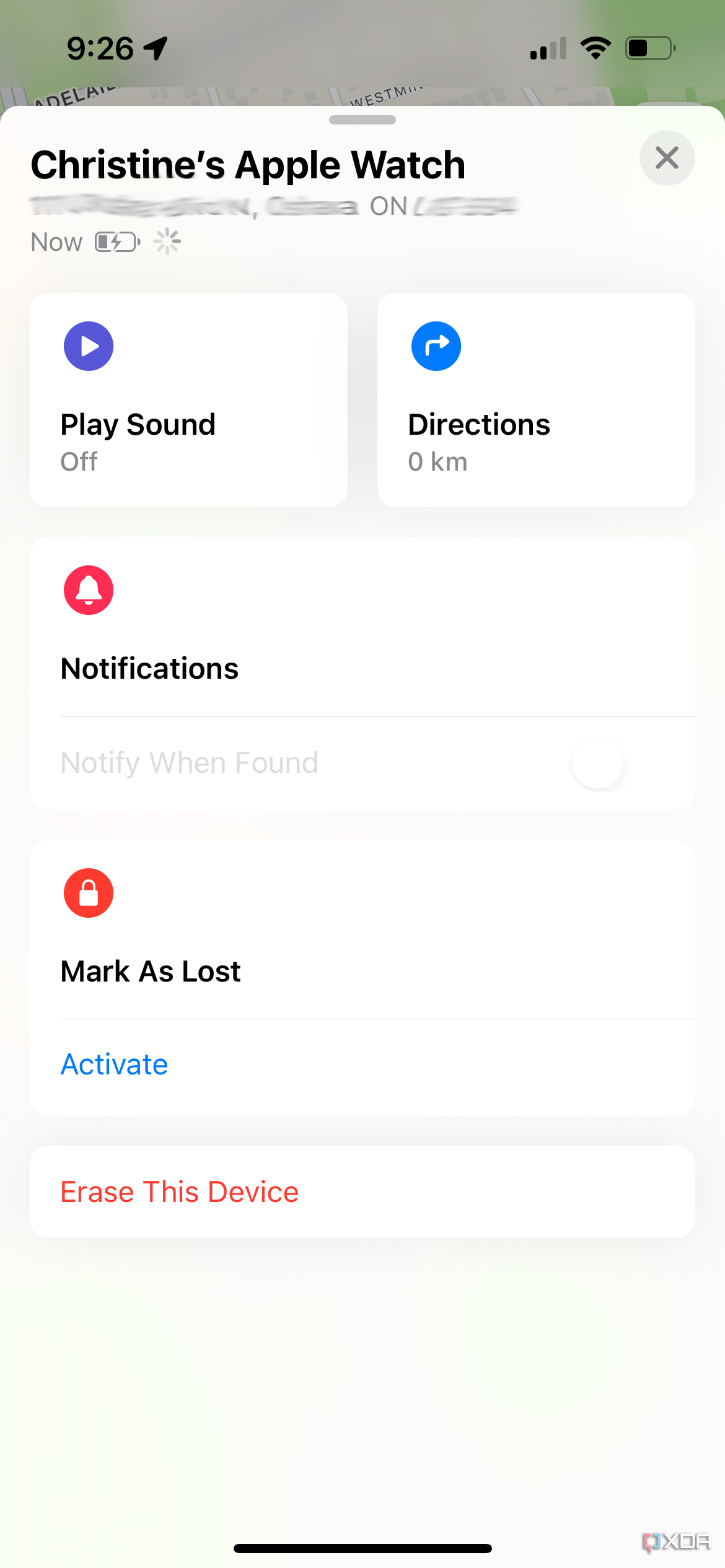This is a detailed screenshot from a mobile phone displaying a pop-up menu overlaying a map application. At the top of the screen, it is 9:26 AM, and location sharing is active. The status bar on the right shows a mobile signal of 2 out of 4 bars, full Wi-Fi connectivity, and a battery level at approximately 40%.

The pop-up menu reveals information pertinent to "Christine's Apple Watch." Although the exact location is blurred out for privacy, black bold font at the top clearly labels the watch's name. Just below this, "now" is displayed in gray font, accompanied by a partially charged battery icon in darker gray and a buffering symbol.

Further down on the left side of the menu, there is a blue circle with a white arrow labeled "Play Sound" in black font, which is currently set to "off" in gray font. To the right, there's another blue circle with an arrow labeled "Directions," with "0 KM" noted in gray font beneath it. The background of the pop-up is a neutral gray, maintaining a clean and focused display.